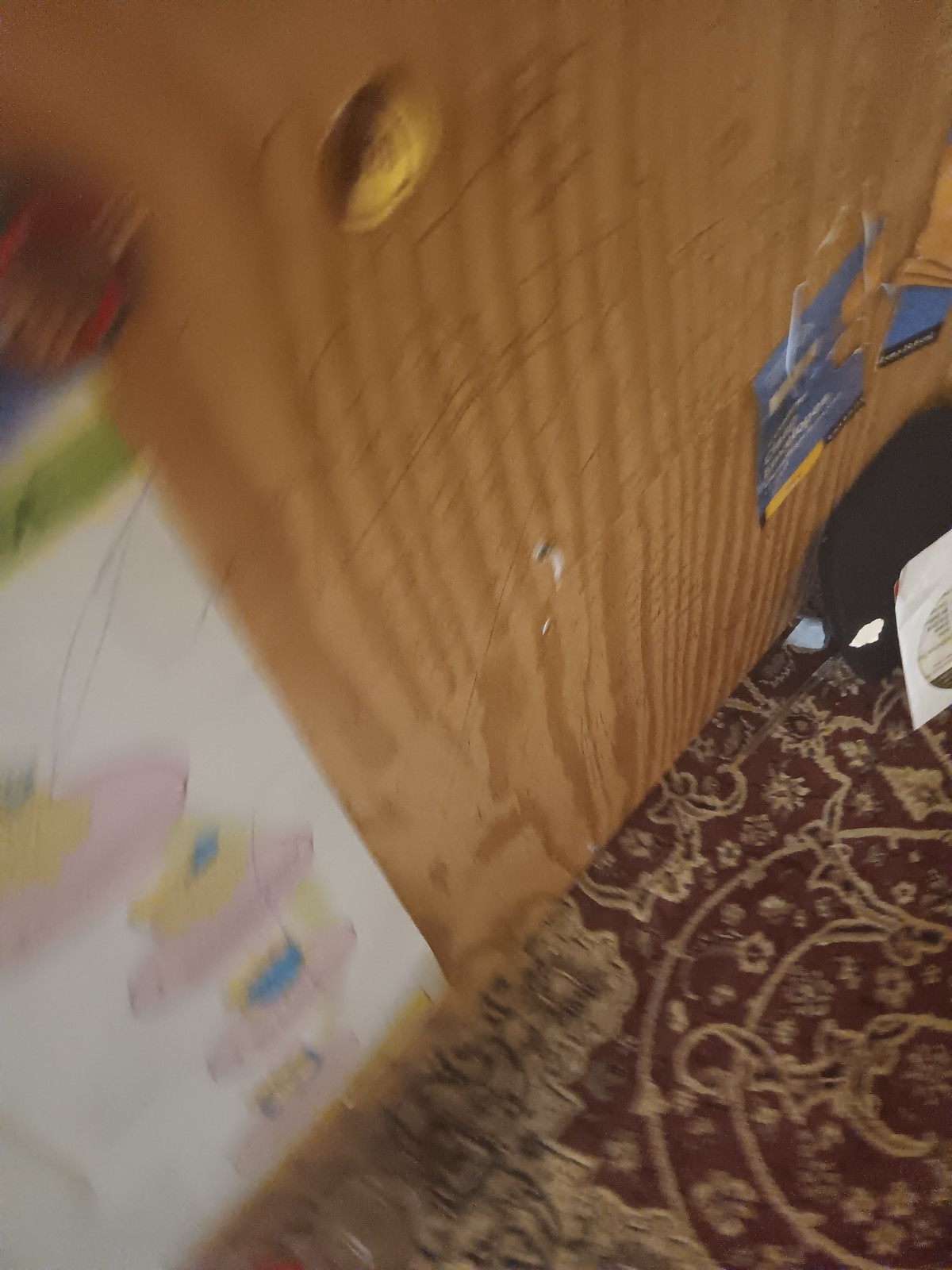The image depicts a sliding door made of bare plywood, not stained or painted, allowing the wood grain to show. The door features a hollowed-out finger pull for sliding it open or closed. There's duct tape on part of the door, possibly where it has been damaged, either kicked or scuffed. This damage is visible along the border of a maroon area rug with gold paisley decorations. Adjacent to the sliding door, there are four pink objects of varying sizes with blue at the top, though their purpose is unclear. Scattered near the door are some loose pieces of paper and possibly a piece of clothing. The lower portion of the image includes part of an oriental-style rug. Affixed to the wall on the left side of the image is a white piece of paper with child-like drawings in pink, yellow, and blue. Positioned towards the top of the photo's center is a lighter circle that could be a knot in the wood. There is also a torn blue sticker-like item on the wall, adding to the texture and detail of the scene.